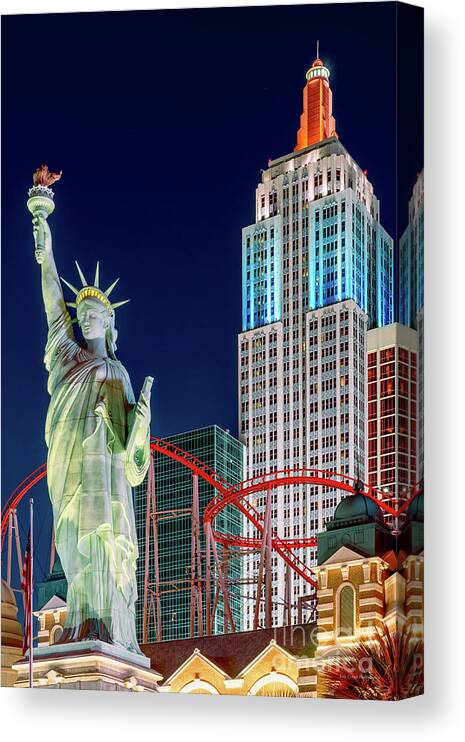The image resembles a portrait-style art piece, created to mimic a photograph printed on canvas. The rectangular canvas prominently features a scene highly reminiscent of Las Vegas. On the left side of the image stands a replica of the Statue of Liberty, complete with its iconic torch. The statue is depicted on a marble pedestal, adding to its majestic presence.

Behind the Statue of Liberty, one can observe various hotel buildings and tall structures that are characteristic of the Las Vegas skyline. A notable feature is a striking red roller coaster that winds its way behind the statue, adding an element of excitement to the scene. Among the buildings, the tallest one catches the eye with its white and blue facade, accentuated by luminous lighting. This building features an orangey tower with a pinnacle at the top, enhancing the vibrant and lively atmosphere of the backdrop.

The sky above is painted in a very dark blue hue, creating a stark contrast with the illuminated structures below. This combined composition might suggest either an actual photograph of Las Vegas or an imaginative, composite image that merges various iconic elements into a whimsical representation.